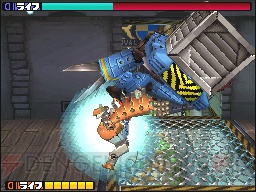A small, blurry screen capture depicting a chaotic scene from a computer game. The central area is dominated by a gray box from which various blue objects are spilling out. Additionally, there's an area marked by distinctive yellow and black caution stripes. A mechanical device with black, brown, and gray elements protrudes from the scene, along with a pair of blades resembling scissors. At the bottom of the screen, a progress bar features six yellow squares alongside the numbers "5, 4, 7" rendered in a stylized font. At the top, the same stylized "5, 4, 7" reappears next to a progress bar that transitions from green to red.